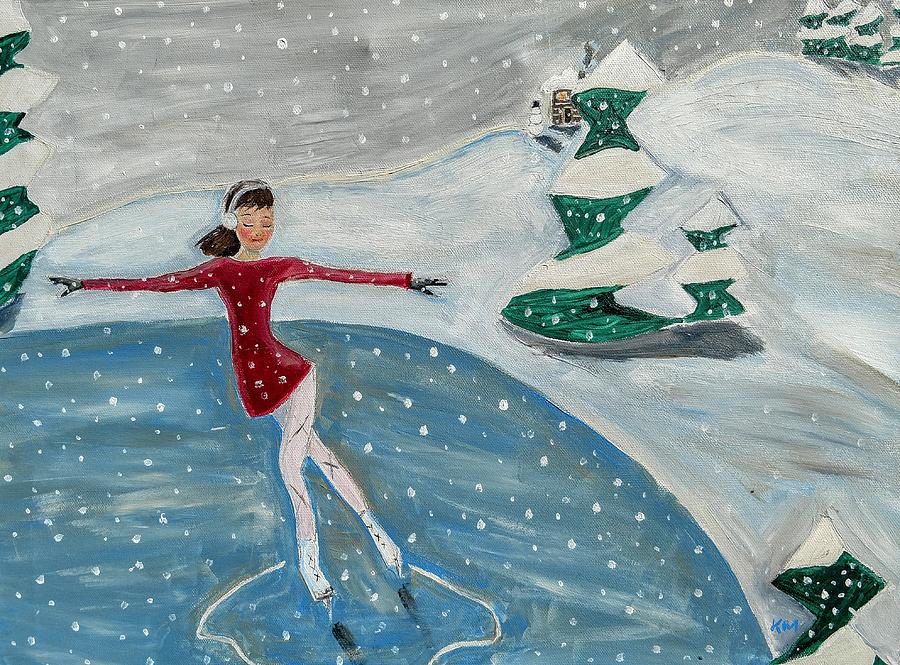In this simple yet charming painting, a female ice skater glides gracefully on a frozen pond amidst a picturesque winter wonderland. She is dressed in a long-sleeve red shirt, white pants, and black ice skates, with white earmuffs snugly covering her ears. Her arms are outstretched in a T-shape as she forms graceful circles on the ice. Snowflakes gently fall from the gray sky, adding a serene ambiance to the scene and creating a flurry effect around her. Surrounding her, green trees dusted with snow frame the landscape, and to the right, a snow-covered hill rises, adorned with snowy plants. In the distant background, a small snowman stands along a path, complete with a hat, and the blurred outline of a house can be faintly seen. The artist, signed as KM, captures the tranquility and beauty of a cold, snowy day.